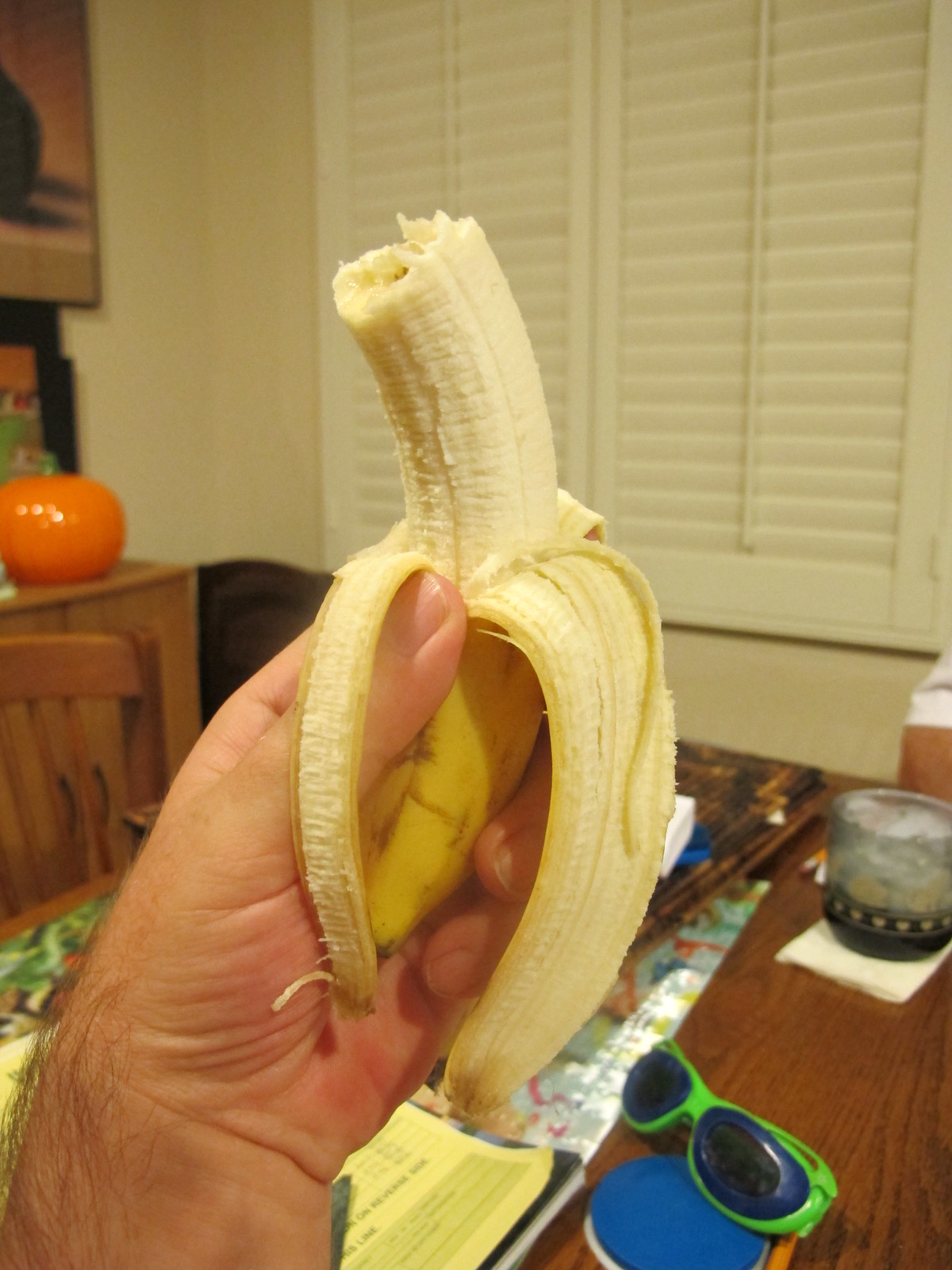In this vividly detailed indoor portrait photograph, a man with light skin is prominently featured in the foreground. His left hand delicately holds a banana that is peeled halfway, revealing the white flesh underneath with a textural detail that indicates at least one bite has been taken. The banana is grasped between his thumb and fingers, showcasing the intricate nature of its partially removed peel.

The background reveals the setting of the photograph, a room inside a house. A wooden table occupies the mid-ground, scattered with various objects that add narrative depth to the scene. A pair of green plastic goggles and a yellow piece of paper with dark print rest on the table. Next to these items sits a squat glass, filled with a light-colored liquid and cooling ice cubes. 

The walls of the room are painted a soothing cream color, enhancing the warm ambiance. Dominating the background is a large louvered shutter, possibly covering a door or window. To the left, a piece of wooden furniture is partially visible. Atop this furniture is a shiny, pumpkin-shaped object, vividly orange with a green stem, bringing a touch of seasonal decor or artistic flair to the photograph.